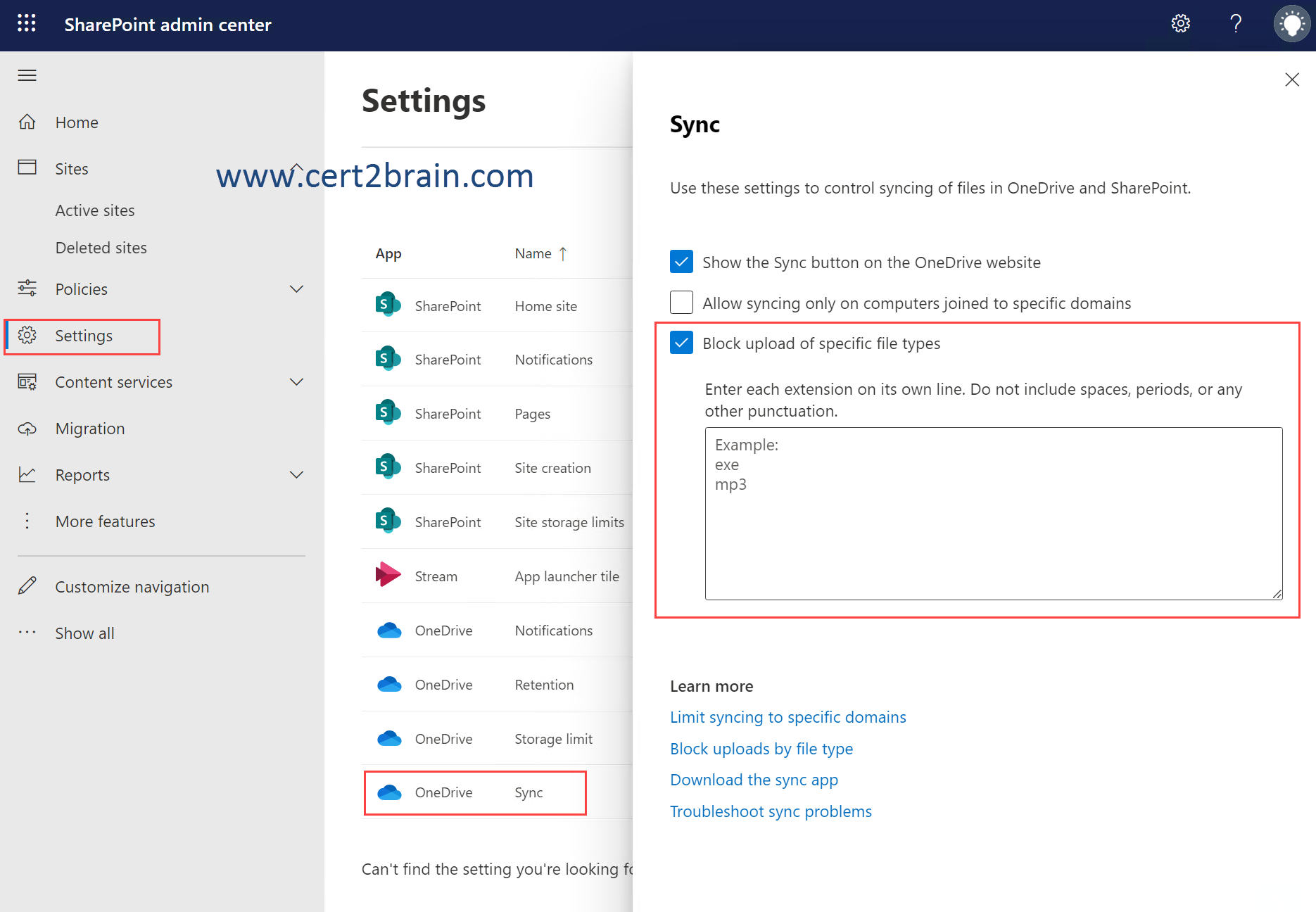**Detailed Description of the SharePoint Admin Center Interface**

The screenshot displays the SharePoint Admin Center, identified by the title at the top. The interface follows a dark blue and white color scheme, characteristic of Microsoft products. Below the header, the layout features three distinct columns, with an additional pop-up sidebar positioned on the right.

The background colors transition from medium gray on the left to light gray and white towards the right. In the first column, notable items are highlighted within a clear rectangle with a red border. Specifically, the 'Settings' option is circled. Within the 'Settings' menu, the 'OneDrive sync' option at the bottom is also circled.

The pop-up sidebar provides detailed instructions regarding syncing settings for OneDrive and SharePoint files. Notably, it features several checkboxes:
1. The first checkbox is checked and labeled "Show the sync button on the OneDrive website."
2. The second checkbox, labeled "Allow syncing only on computers joined to specific domains," is unchecked.
3. The third option, which is checked and emphasized with a red outline, is "Block upload of specific file types." Instructions indicate that users should enter each file extension on a new line without including spaces, periods, or any other punctuation. Examples given include "exampleexe" and "examplemp3."

Near the bottom of the pop-up, there are additional links related to synchronization:
- Learn more
- Limit syncing to specific domains
- Block uploads by file type
- Download the sync app
- Troubleshoot sync problems

This detailed depiction captures the interface elements and user instructions for managing OneDrive sync settings in the SharePoint Admin Center.